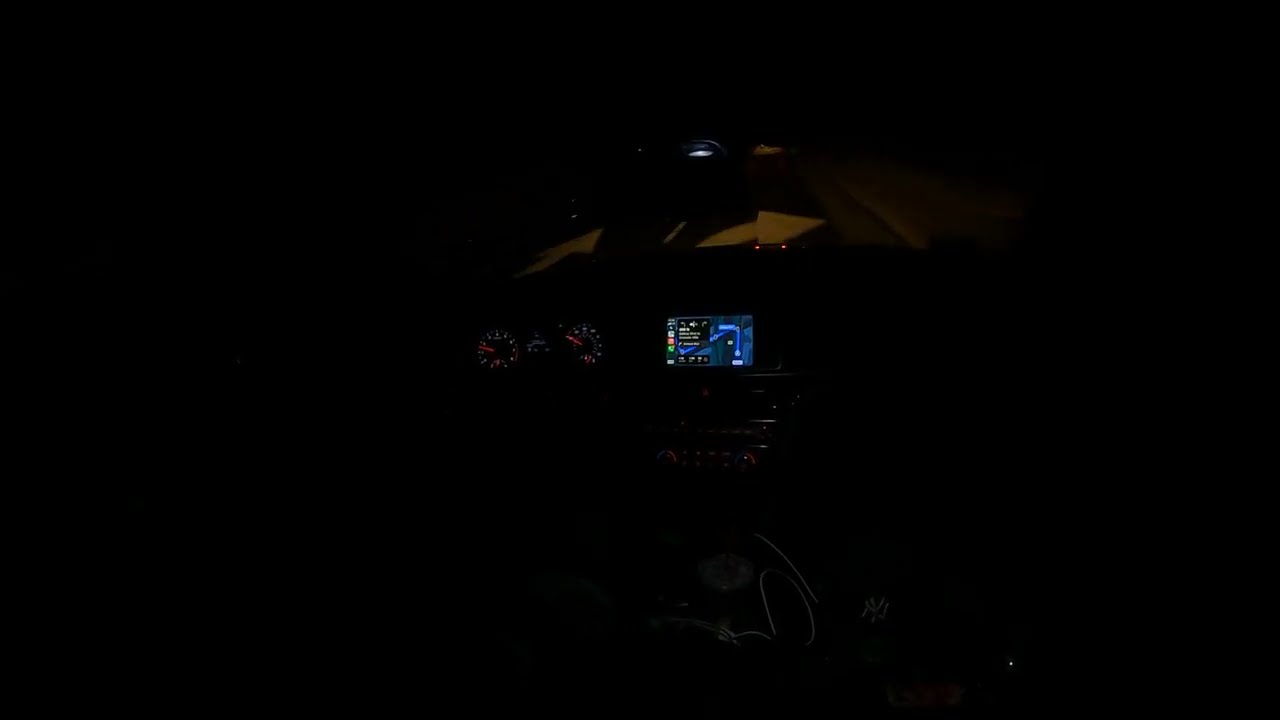The image is predominantly dark, seemingly taken from the interior of a car at night. The majority of the photo is black, but some illuminated details stand out. At the center is a lit speedometer displaying bright red and white numbers with a red needle. Nearby, a lit screen emits a mix of blue, green, red, and white colors, resembling a car radio or a dashboard menu interface. 

Below the main screen, faint hints of dials and buttons are discernible, likely for temperature control, and a barely visible white cord suggests a phone charger. Two circular gauges, probably the speedometer and an odometer, have black backgrounds with white numbers and red needles. Beyond the gauges, there appears to be a window, through which parts of a road can be seen. There are dimly visible white arrows on the road: one pointing straight ahead and another curving to the right. The interior setup includes a few push buttons and touch screen controls, enhancing the idea of a comprehensive car dashboard illuminated amid the darkness.